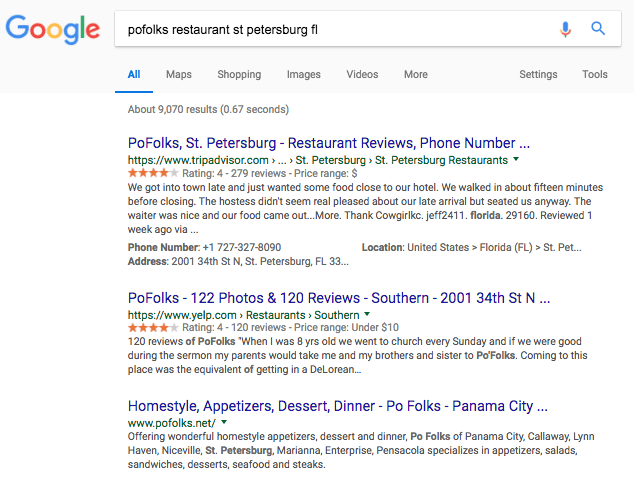A screenshot of Google search results for "Poe Folks Restaurant, St. Petersburg, Florida" is displayed, with the Google logo prominently displayed in the upper left corner of the page. A gray bar runs horizontally beneath the logo, containing a white search box pre-filled with the search query. To the right of the search box are the microphone icon, allowing voice search, and the magnifying glass icon, which indicates the search function.

Below the search bar is a horizontal menu with various search categories: "All" (highlighted in blue and underlined), "Maps," "Shopping," "Images," "Videos," "More," "Settings," and "Tools." The page indicates approximately 9,070 search results retrieved in 0.67 seconds.

The top search result is highlighted in blue text and reads "Poe Folks St. Petersburg restaurant reviews, phone number, ..." provided by TripAdvisor. The URL that follows is partially visible, starting with "https://www.tripadvisor.com..." and includes drop-down options for St. Petersburg Restaurants. Summary details of the restaurant include a rating of four out of five stars based on 79 reviews, and a price range indicated by a single dollar sign. The brief snippet from one review mentions an experience where the visitors arrived about 15 minutes before closing, noting the hostess's less-than-enthusiastic reaction to their late arrival.